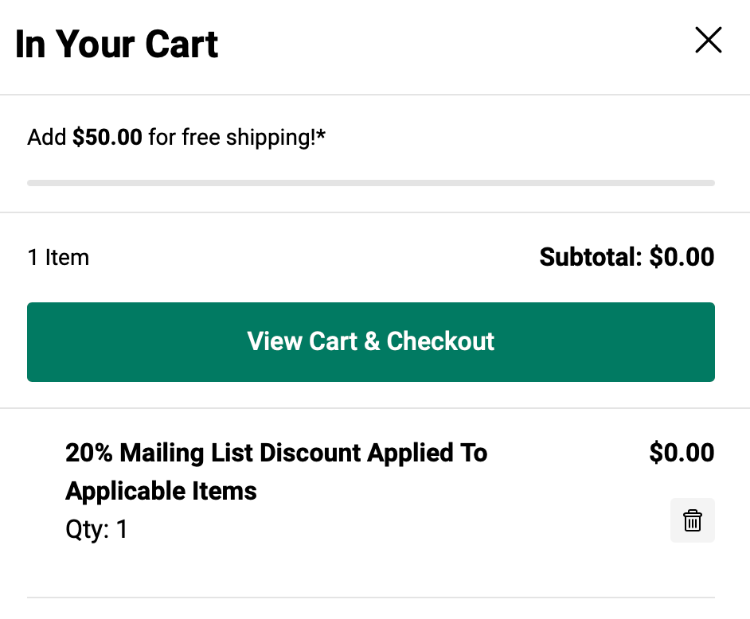The image is a partial screenshot of an online shopping cart page. The top of the page displays the text "In Your Cart," although the specific store name is not visible. Below this section, there's a notice highlighting that the customer needs to add $50 worth of items to qualify for free shipping.

The cart currently contains one item, listed at a cost of $0. A teal-colored "View Cart Checkout" button is prominently displayed, allowing users to proceed with their purchase. Additionally, the cart mentions a 20% discount applied from a mailing list, which is reflected as $0 since the item already costs nothing. The cart summary also includes options to adjust the quantity and a delete button for removing the item. At the top right corner of the page, an 'X' is available for customers to exit the cart view.